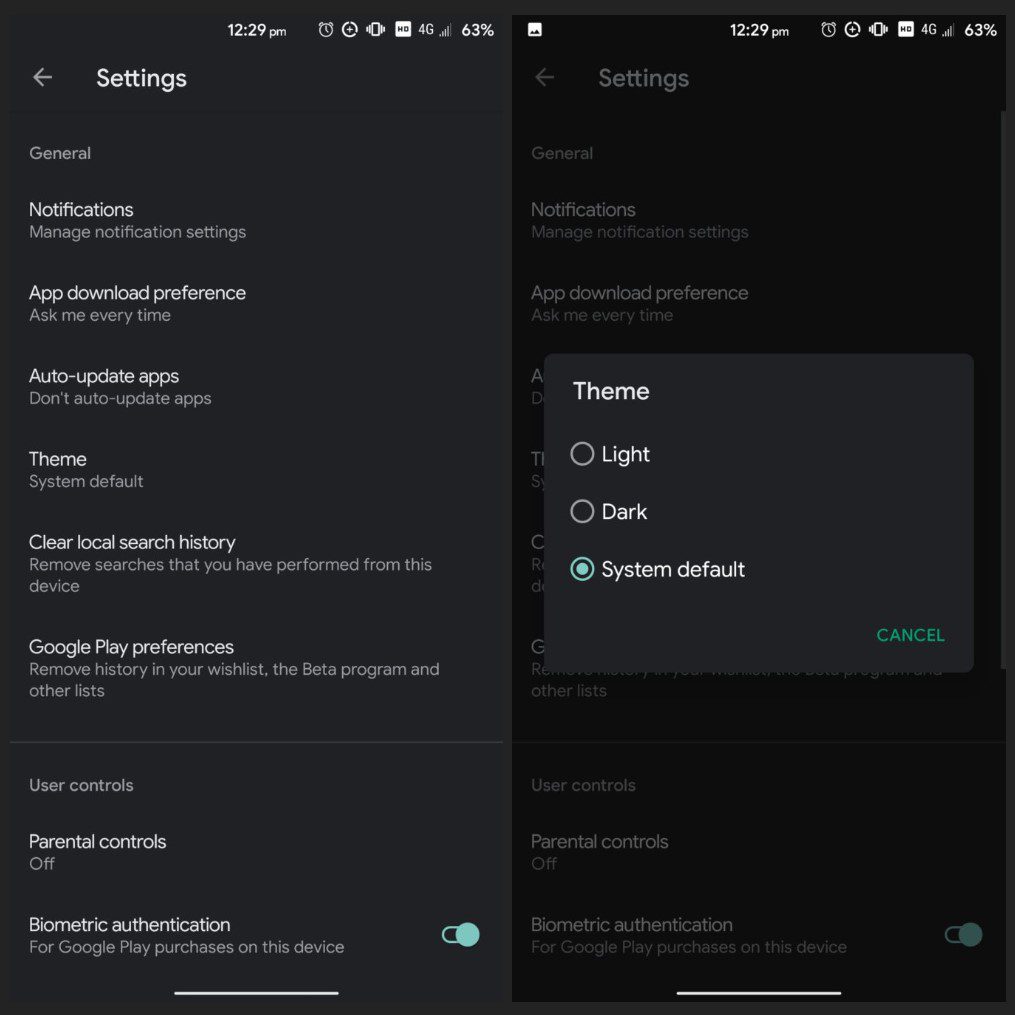This image features a black background with two cell phone layouts displayed side-by-side. Both layouts show identical status bars at the top, with the time "12:29 p.m." on the left, followed by several icons: a clock, a plus sign within a circle, an exclamation mark within a circle, a white box labeled "4G," a cell signal strength icon, and a battery icon indicating 63% charge.

The left layout has a grayer color scheme compared to the more distinct colors of the right layout, suggesting a possible difference in themes or settings. The right layout features an additional open box overlay labeled "Theme," which includes options for "Light," "Dark," "System Default," and "Cancel." The option "System Default" is currently selected. Overall, the two layouts appear to be mirror images except for this thematic overlay on the right.